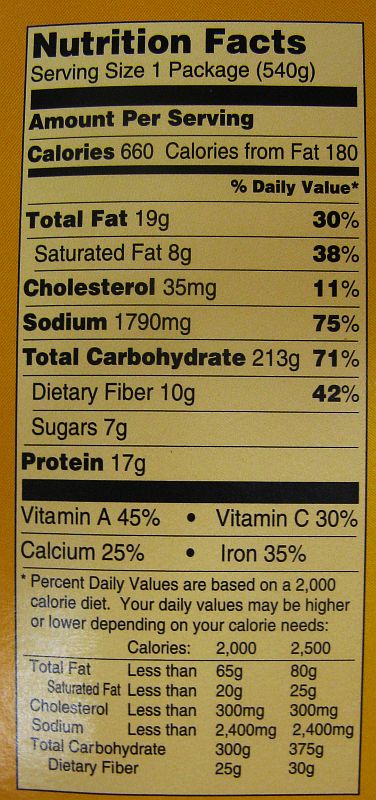This is a detailed photograph of the Nutrition Facts label on the back of a food package. The label is prominently displayed with large bold text at the top reading "Nutrition Facts." The label design is classic, featuring black text on a white background, with accents in a light brown or cream color, and surrounded by a yellow border. At the top, it specifies the serving size as "1 Package" (540g). Below, it provides a detailed breakdown of nutritional information: 

- Calories: 660 (with 180 calories from fat)
- Total Fat: 19 grams (30% of daily value)
- Saturated Fat: 8 grams (38% of daily value)
- Cholesterol: 35 mg (11% of daily value)
- Sodium: 1790 mg (75% of daily value)
- Total Carbohydrates: 213 grams (71% of daily value), including 10 grams of dietary fiber (442% of daily value) and 7 grams of sugars.
- Protein: 7 grams

Additionally, it lists the percentage of daily values for vitamins and minerals: 

- Vitamin A: 45%
- Vitamin C: 30%
- Calcium: 25%
- Iron: 30%

The bottom section notes that these daily values are based on a 2000 calorie diet, with a disclaimer that individual caloric needs may vary. Overall, the photo focuses solely on the nutrition label, providing no further indication of what the product might be.